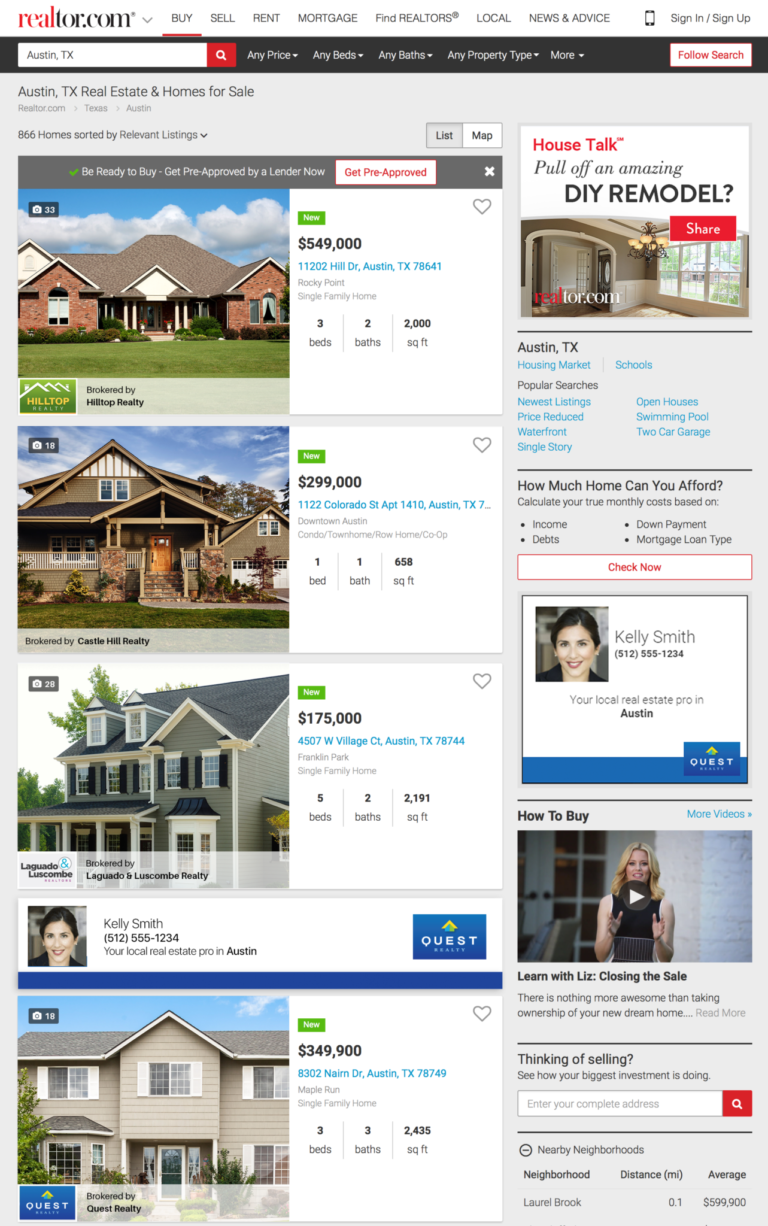This image is a detailed screenshot from Realtor.com featuring homes for sale in Austin, Texas. At the top of the page, there's a navigation banner offering various options such as Buy, Sell, Rent, Mortgage, Find Realtors, Local News, and Advice, with the 'Buy' option selected. Just below the banner is a search bar where "Austin, Texas" is entered, accompanied by additional filters for price, beds, baths, property type, and more.

Immediately underneath, the section titled "Austin, Texas real estate and homes for sale" begins with four prominent listings:

1. **New Listing**: A brown, single-family home with a brown roof at **11202 Hill Drive, Austin, Texas**. This property, priced at **$549,000**, features 3 bedrooms, 2 bathrooms, and encompasses 2,000 square feet. It is brokered by Hilltop Realty.

2. **Second listing**: A dark green, two-story house located at **1122 Colorado Street, Apartment 1410, Austin, Texas**. Listed at **$299,000**, this home offers 1 bedroom, 1 bathroom, and spans 658 square feet.

3. **Third listing**: Another greenish, two-story single-family home situated at **4507 West Village Court, Franklin Park, Austin, Texas, 78744**. This property is listed at **$175,000** and includes 5 bedrooms, 2 bathrooms, over 2,191 square feet.

4. **Fourth listing**: A beige-colored home at **8302 Nairn Drive, Austin, Texas, 78749**. Priced at **$349,900**, this house has 3 bedrooms, 3 bathrooms and covers 2,435 square feet.

On the right-hand side of the screen, there is additional information about the Austin, Texas housing market, providing further insight into the local real estate trends.